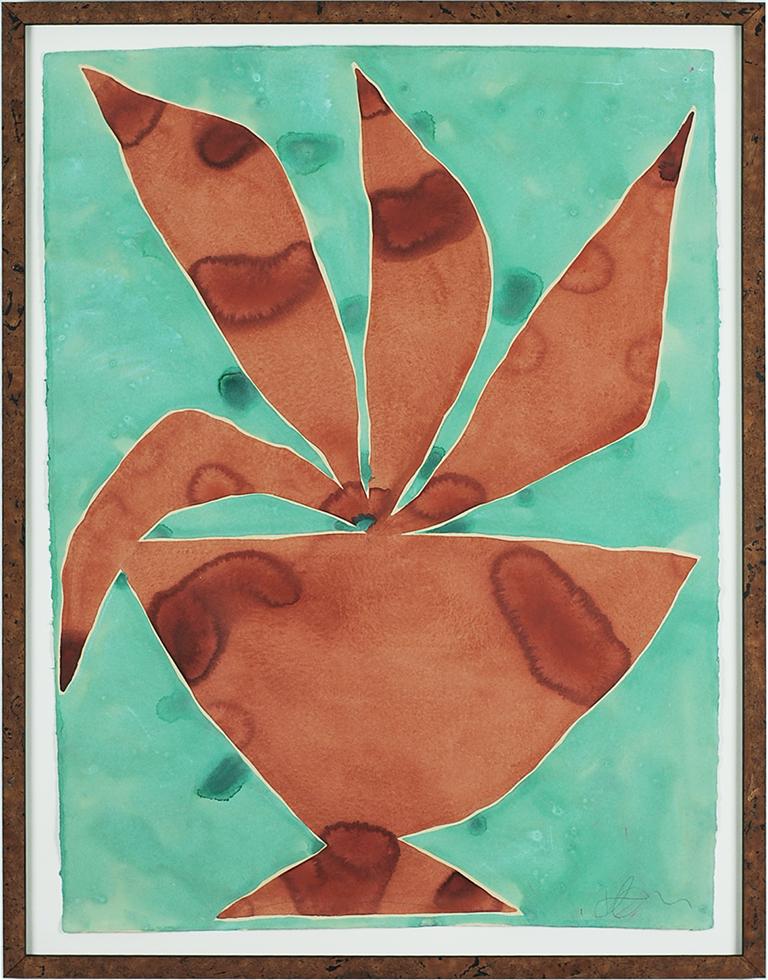This image captures a digital photograph of a framed abstract painting, housed in a large, dark brown wooden frame with a white inner border. The background of the painting is a warm light green, featuring mixed shades of darker green circular areas, along with small white and light green speckles. Central to the image is a peculiar, V-shaped form that could be interpreted as either a rudimentary flower pot or a strangely shaped head. This central shape is predominantly brown with dark brown splotches and features four protruding leaf-like elements, which also have dark circular areas. There is a faint, indecipherable signature in the bottom right corner of the painting. Overall, the piece combines elements of green, brown, and white, contributing to its abstract and somewhat ambiguous appearance.